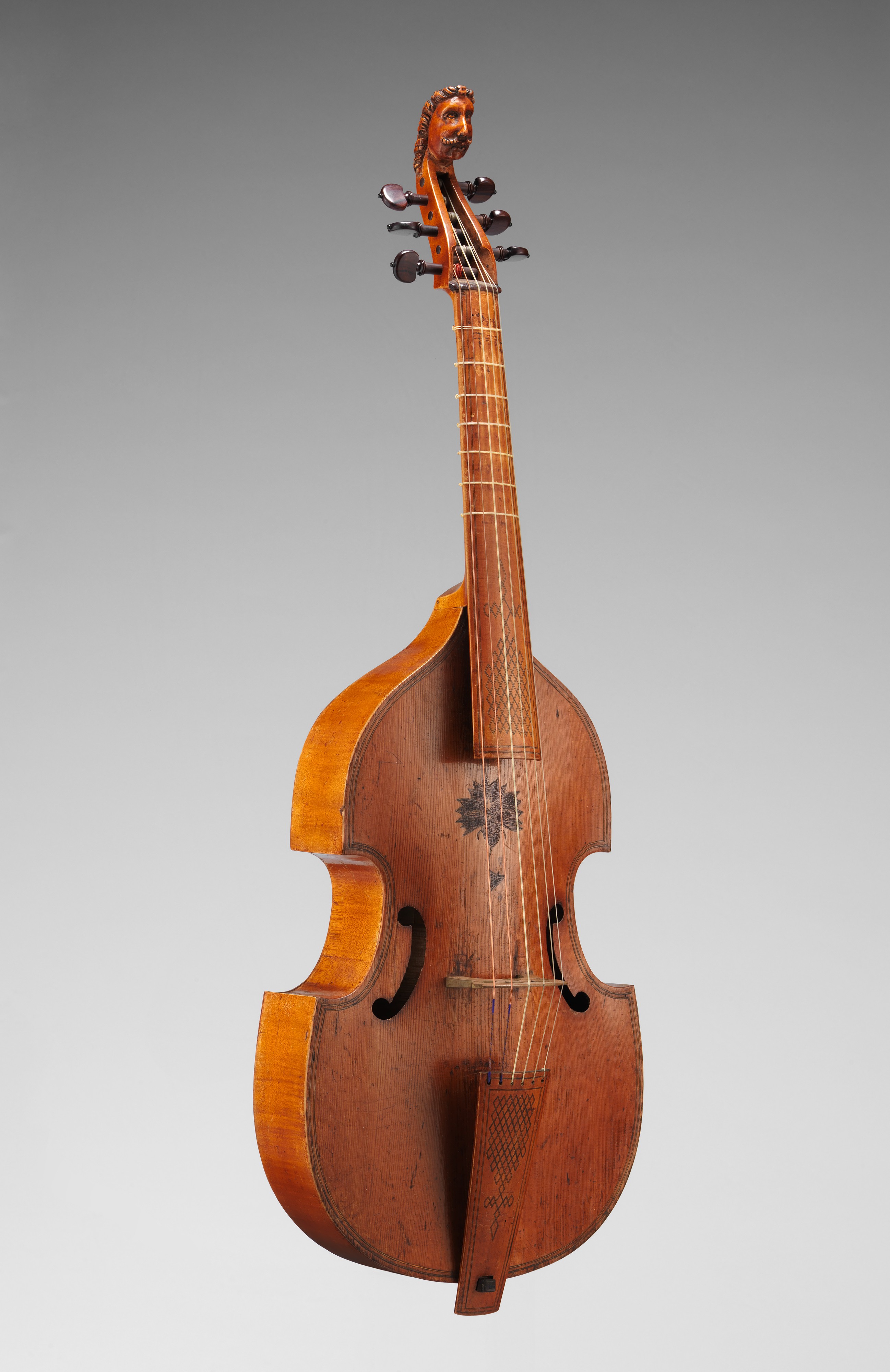This image showcases a unique and beautifully crafted antique stringed instrument that resembles a cello, violin, or bass in its classic contours, but with distinctive features setting it apart. Notably, it has six strings, unlike the traditional four-string setup of cellos, violins, and basses. The instrument is made of plain, high-quality wood and styled with narrow shoulders, a swooping design, and a tailpiece. It features a bridge and frets on the fingerboard, with keyholes positioned unusually on either side of the bridge. The fingerboard is adorned with intricate etching that appears to be a sunburst pattern, and the tuning pegs, six in total, are wooden. A remarkable detail is the carved head of a man at the top of the stem, adding to its ornate and possibly considerable value. This rare piece reflects exquisite craftsmanship and has been well-preserved, suggesting it might be hundreds of years old. The background of the image is plain gray, emphasizing the instrument's elegant and detailed artistry.